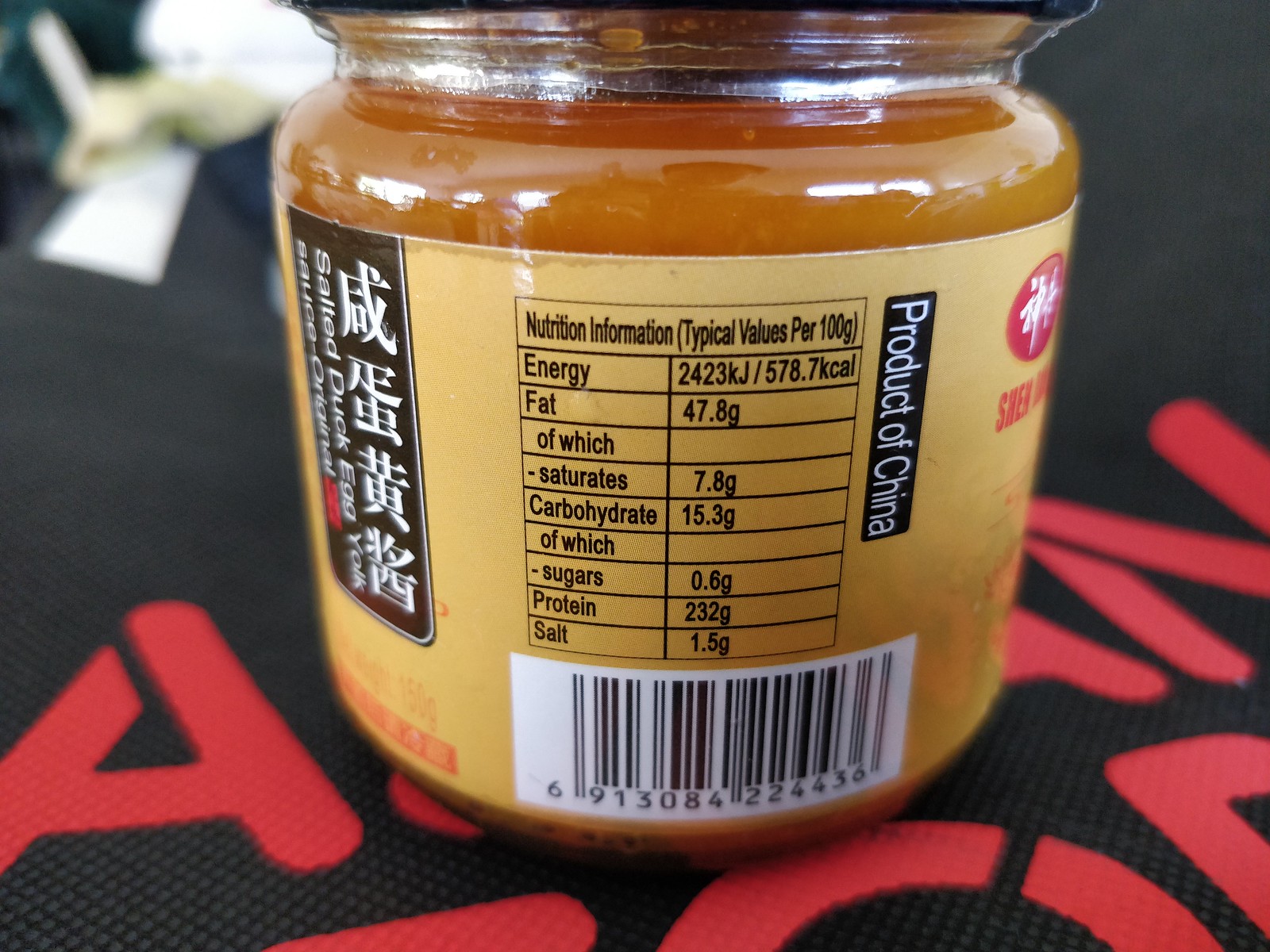This detailed close-up photograph features a small, clear glass jar, roughly the size of a baby food jar, containing an amber-colored sauce described as salted duck egg yolk sauce. The jar is topped with a tan label bearing intricate details. On the left side of the label, Chinese symbols are visible above the text that reads "salted duck egg yolk sauce original." The center of the label prominently displays nutritional information, which is outlined in a table format with black font, highlighting values per 100 grams: energy 2023 kilojoules (578.7 kilocalories), fat 47.8 grams (of which saturates 7.8 grams), carbohydrates 15.3 grams (of which sugars 0.6 grams), protein 232 grams, and salt 1.5 grams. Adjacent to the nutritional table, the words "product of China" are printed in white font within a black rectangular box, and a black and white UPC barcode appears below the nutritional information. The jar is placed on a black surface adorned with red writing, although only hints of this writing are visible.